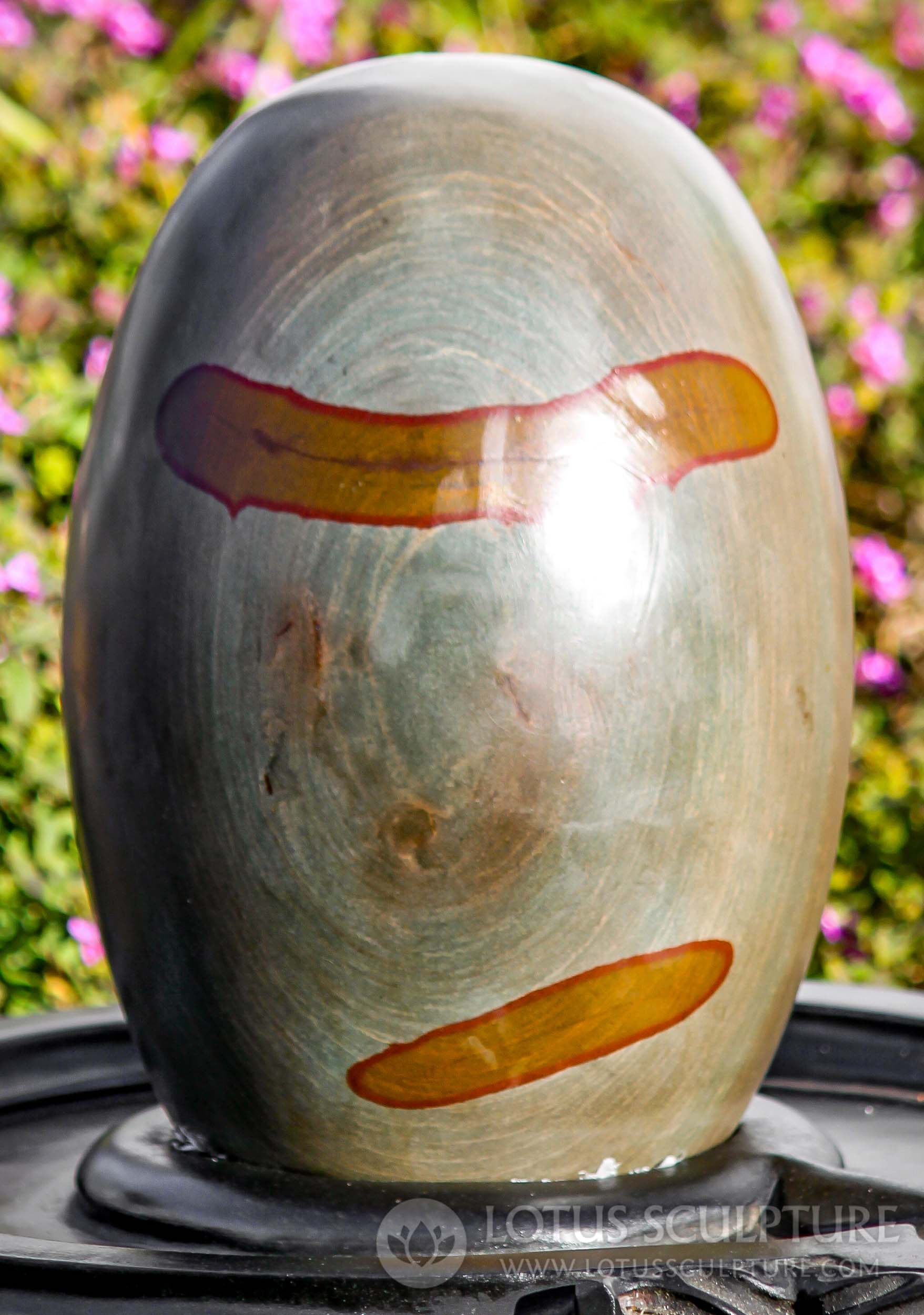The image features a close-up of an art piece, most likely a pottery sculpture, with an egg or oval-like shape. This sculpture is primarily gray with a polished, shiny, and reflective surface that exhibits thin, circular lines or swirls converging at the center. Two distinguishable rectangular, orange-yellow strips with red outlines are present—one above the center and the other below, albeit shorter. The sculpture appears to be set on a black display platform atop a table. The background is blurred, revealing green bushes with pink flowers, providing a contrasting natural backdrop. Additionally, there's a watermark in the bottom right corner that reads "Lotus Sculpture" with the website "www.lotussculpture.com" underneath.